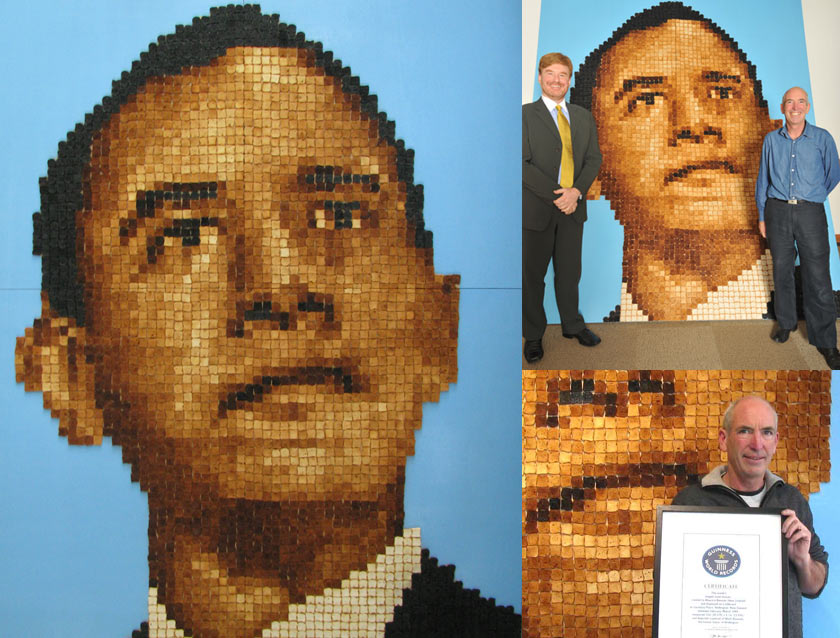The composition is a triptych collage featuring a pixelated portrait of Barack Obama, heavily utilizing a mosaic aesthetic composed of small light brown, dark brown, white, and black squares. The largest image, situated on the left, showcases Obama in a hopeful gaze upward, dressed in a white shirt and black suit coat against a blue background, reminiscent of his appearance around his first presidential campaign. The right-side of the collage includes two smaller, vertically-stacked photographs. The top picture mirrors the large Obama portrait but with two men standing beside it: the man on the left is in a dark suit, gold tie, blue and white shirt, and smiling, while the man to the right dons black slacks and a blue button-up shirt. Both men are white. The bottom right image zooms in on another white man, casually dressed in a black and gray jacket, holding a framed plaque resembling a Guinness World Record certificate, suggesting he might be the artist behind the creation. This carefully crafted collage captures both the intricate detail of the mosaic portrait and the context of its display.